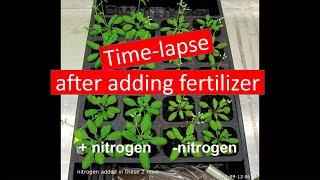This image appears to be a grainy screenshot, potentially from a YouTube video or TikTok, illustrating a time-lapse experiment on plant growth after adding fertilizer. The image within the image is framed by black borders on either side. At the top of the inner image, a red text box with white letters reads, "Time-lapse after adding fertilizer." Below this, there's a black tray containing young, green plants in various stages of growth. The tray is segmented, allowing for multiple plants to grow in small, separate areas of soil. Distinctively, the left side of the tray is labeled “+ nitrogen” and the right side “- nitrogen,” with visible differences between the two. The plants on the "+ nitrogen" side appear larger and more robust compared to those on the right. The fine print at the very bottom of the image mentions "nitrogen added" but is otherwise illegible.